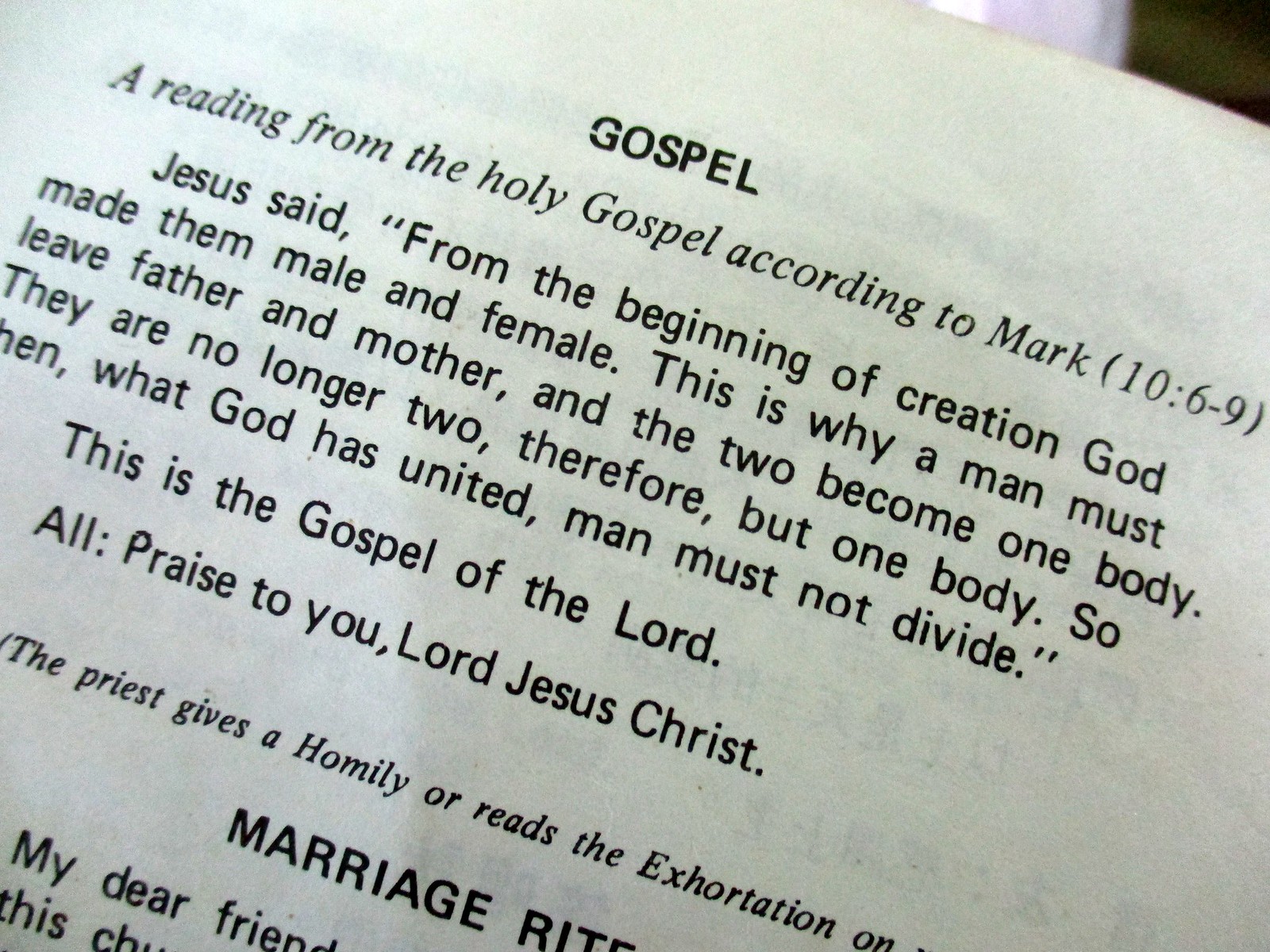The image is a photograph of a diagonally oriented page from a church book, possibly a ceremonial booklet used in religious services. The white page, featuring black text, fills the entire frame. The text begins with the title "GOSPEL" in bold block letters, followed by "A Reading from the Holy Gospel According to Mark (10:6-9)" in italics. The passage reads: "Jesus said, 'From the beginning of creation, God made them male and female. This is why a man must leave father and mother, and the two become one body. They are no longer two, therefore, but one body. So then, what God has united, man must not divide.'" A concluding line states, "This is the Gospel of the Lord," with the response instruction "All: Praise to you, Lord Jesus Christ." At the bottom of the page, partially cut off, there is a note in italics: "(The priest gives a homily or reads the exhortation on...)." Below this, the page appears to begin a new section titled "MARRIAGE RITE" with an introduction starting "My dear friend, this..." The setting is likely indoors, potentially within a church.